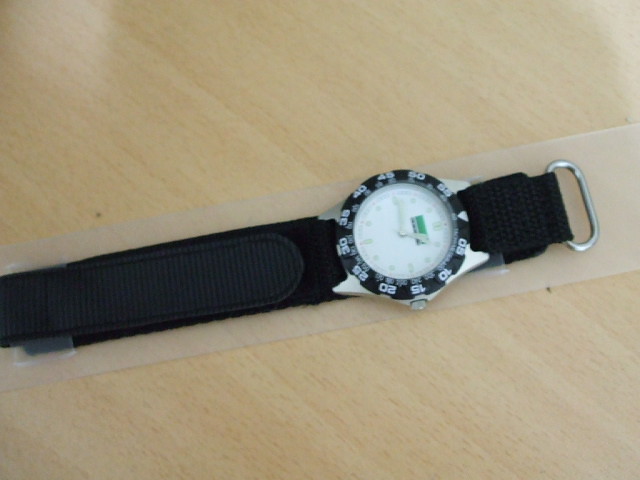A wristwatch is meticulously placed on a light-colored wooden tabletop, oriented diagonally from the bottom-left corner to the top-right corner. The black band of the watch stretches from the 8 o'clock position on the left to the 3 o'clock position on the right. The watch band lies flat, seemingly still attached to a slightly translucent plastic strip underneath it. On the left side of the watch, the straight portion of the band, designed with holes for clasping, is visible. On the right side, at the 3 o'clock position, a steel oval loop is noticeable, intended for threading the band through to secure it.

At the center of the composition is the watch's face, angled on its side with 9 o'clock pointing upwards and 3 o'clock downwards. The dial of the watch is white, complemented by light-colored hands. Encircling the dial, a black bezel featuring bold white numeral increments at 5-second intervals (5, 10, 15, 20, etc.) enhances the watch’s readability. Positioned at where 12 o'clock would be, a small, distinct arrow provides a reference point on the bezel.